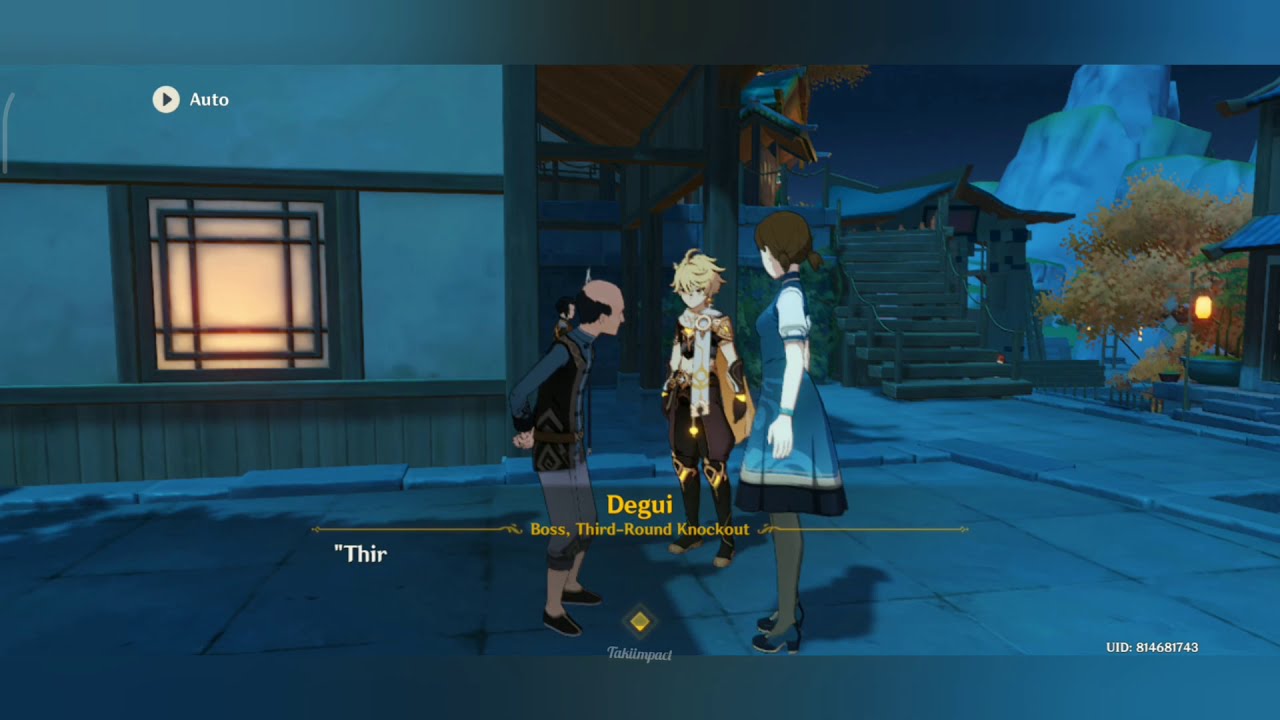The image appears to be a nighttime screenshot from an anime-style role-playing video game. It shows a stone square within a town or living quarters, complete with several illuminated buildings in the background. The scene features three central characters: an older, small, balding man with a ponytail who is hunched over and seemingly addressing a younger, very stylized anime character resembling a Pokemon trainer, sporting blonde hair and dressed in an ornate, heroic gold, white, and black outfit. Beside them is a girl or woman in a blue and white dress, who is closer to the viewer and turned towards the blonde-haired character. In the backdrop, there is a lit house window, a distant hanging lantern, trees, and towering mountain or ice boulders. The game interface elements include a play button labeled “Auto” in the top-left corner and dialogue text at the bottom saying "De gui, boss, third round knockout." A UID "814681743" is displayed at the bottom right. The colors in the scene are predominantly blue, yellow, black, gray, brown, green, and orange. The overall aesthetic places the viewer in an interactive and vibrant anime-inspired RPG world.